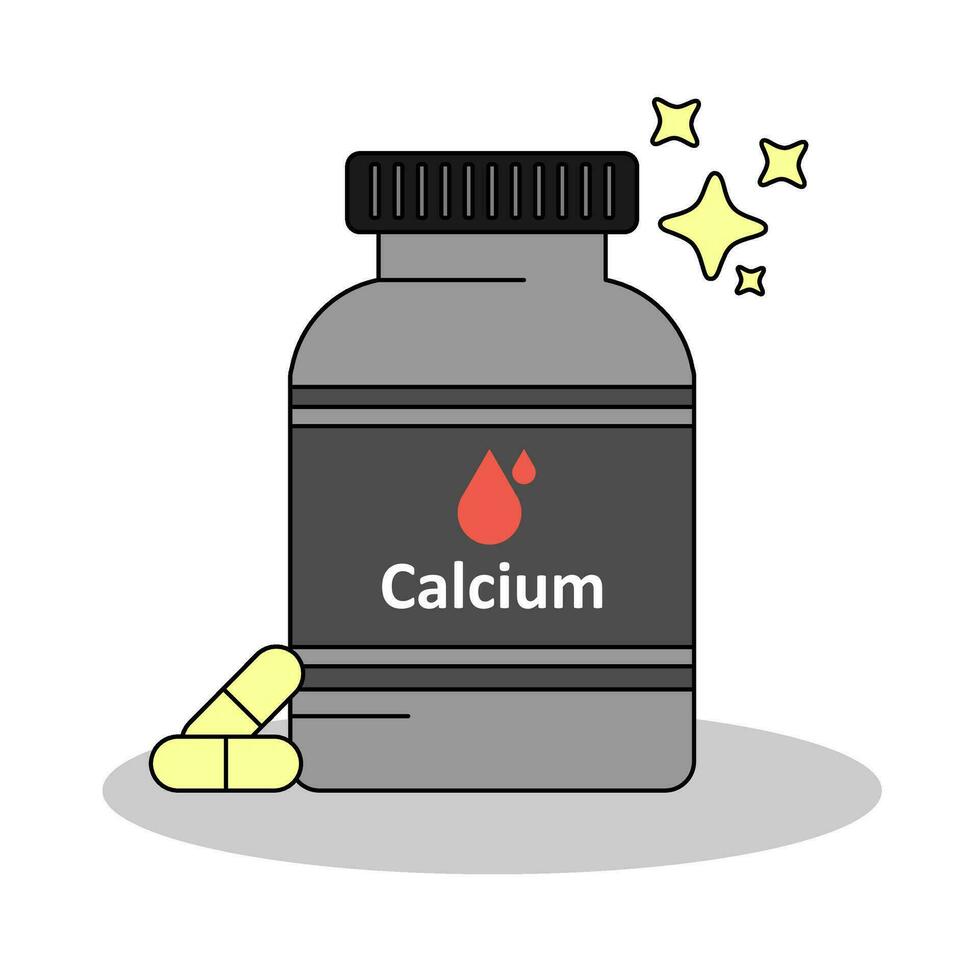This image is a simplistic computer-drawn illustration of a light gray bottle of calcium supplements with a narrow neck and a black screw cap. The bottle features a dark gray label with the word "calcium" written in white font below two red droplets, one larger than the other. To the left of the bottle, two light yellow gel capsules are positioned, one leaning against the bottle and the other lying flat. On the top right side of the image, there are four cartoonish, yellow star shapes. The bottle is placed on an oval, light gray shaded area on a blank white background. The illustration is straightforward with color fill and lacks 3D shading, focusing on clear, clean lines and simple color contrasts.